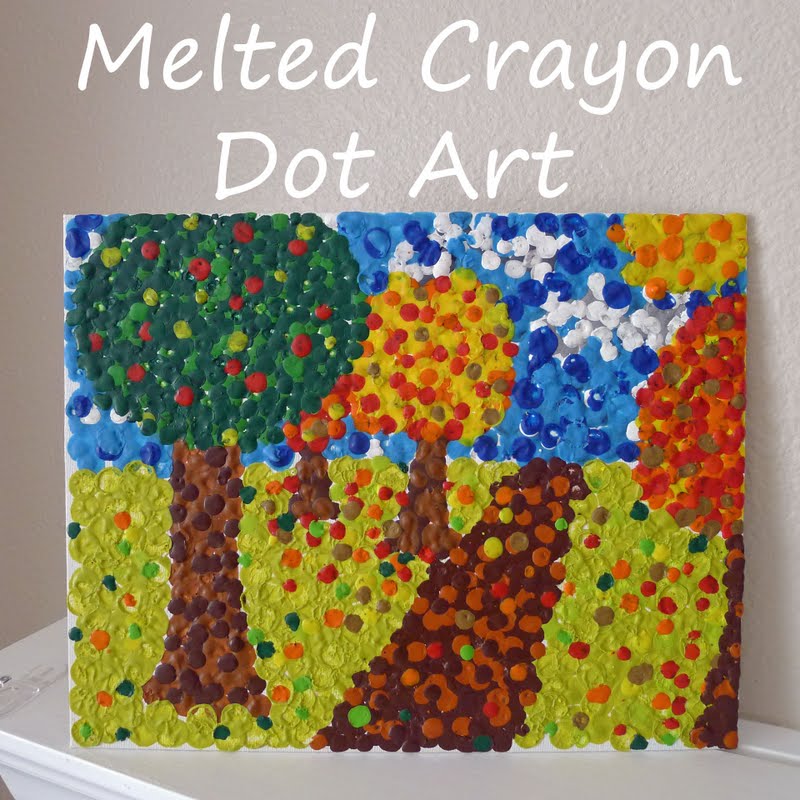This large, perfectly square piece of artwork, titled "MeltedCrayon.art," leans against a textured wall that appears beige or light gray. Positioned on a white wooden shelf, the artwork prominently features the text "Melted Crayon Dot Art" at the top in large white letters. The intricate scene is crafted from melted crayon dots, creating an almost pointillist effect. The artwork depicts multiple trees in a colorful landscape: a large tree on the left with a brown trunk and a canopy of green, red, and bright green dots, a smaller tree in the middle with vibrant yellow, red, and orange leaves, and another tree partially visible on the far right. A pathway with varying shades of brown and some blended green and red hues winds through the scene. The sky is represented by different shades of blue with white dots suggesting clouds. The green ground is dotted with colors indicating fallen leaves or fruit, contributing to the overall leafy effect. The detailed dot work gives the impression of a vivid, dynamic landscape.